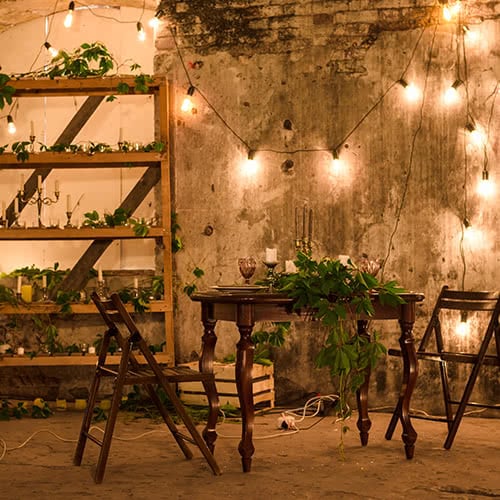The photograph captures a cozy, rustic indoor setting, reminiscent of a room inside a barn or shed, perfect for an intimate dinner for two. The backdrop features a painted-over brick wall with warm, glowing string lights draped across it, casting a gentle ambiance. Centrally positioned in the room, there is a dark-colored, antique-looking wooden table adorned with trailing plants, glass goblets, and several candles in stands. Two wooden folding chairs, devoid of cushions, flank the table, reinforcing the rustic charm. On the left side, a wooden shelving unit holds an assortment of candles—slender white ones, a thicker yellow candle, and a three-candle holder—alongside decorative ivy. A wooden milk crate can be spotted in the background, adding to the room’s rustic appeal, while cords trail discreetly on the floor, hinting at the space's functional aspects. The combination of these elements creates a serene and inviting atmosphere, ideal for a quiet evening.